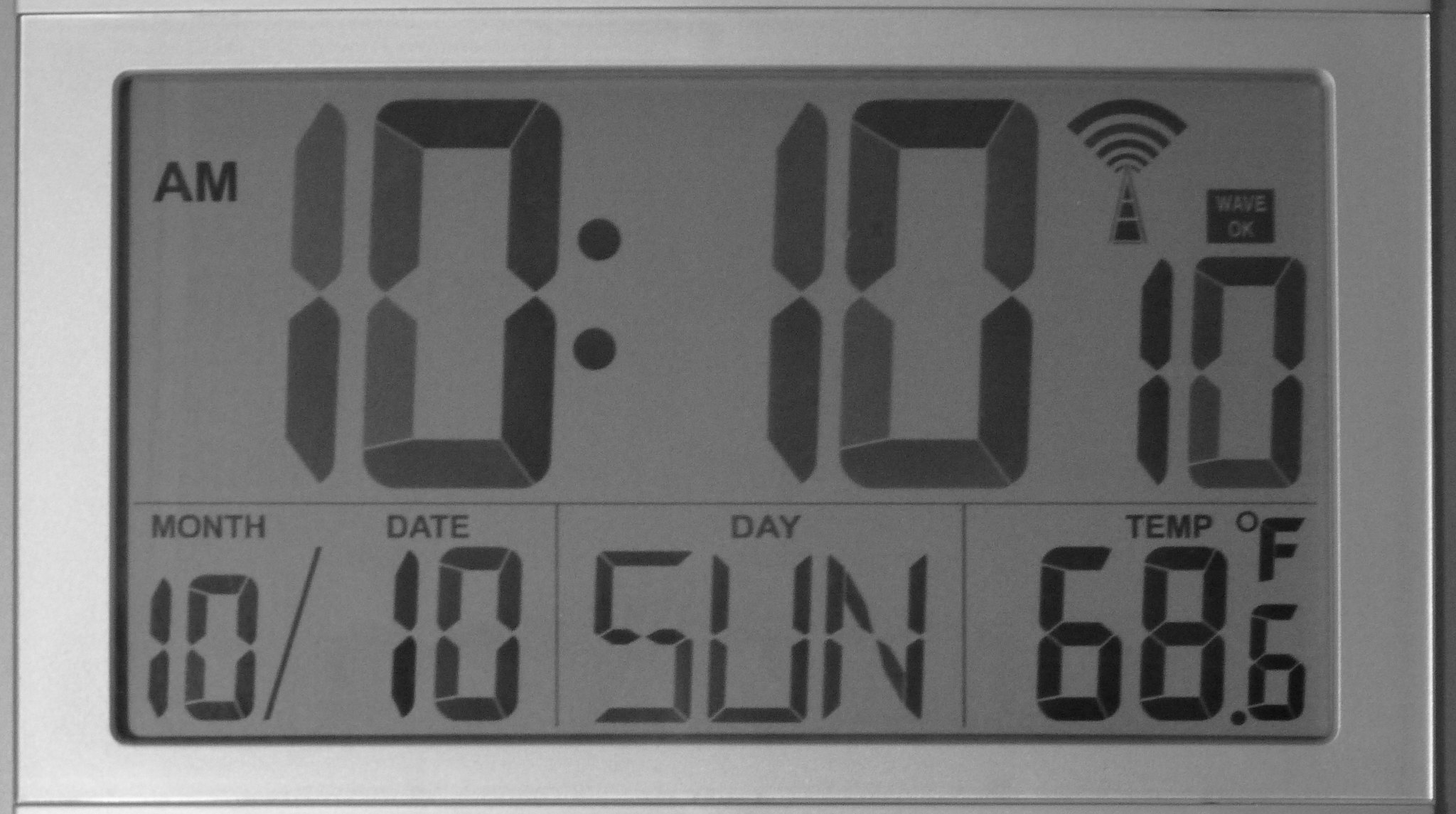This close-up image showcases a rectangular, silver-painted alarm clock, with most of its front occupied by the clock display. The current time is prominently featured at the top in large black numerals, reading 10:10:10 a.m. set against a gray background. Below the time display, there are three smaller sections providing additional information: the date, which is October 10th, the day of the week, which is Sunday, and the current temperature, which is 68 degrees Fahrenheit. The detailed layout makes it easy to read and provides comprehensive information at a glance.